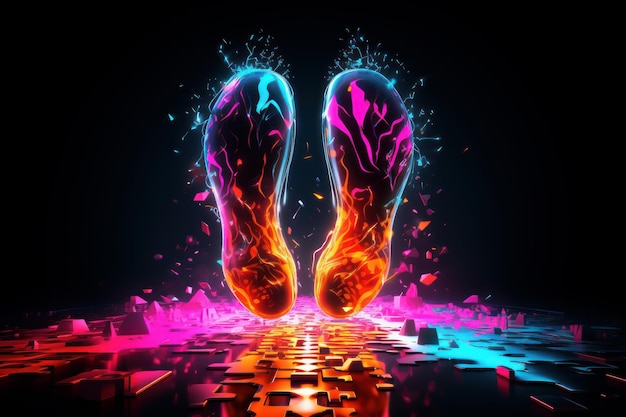In the center of a black background, a vibrant and futuristic 3D illustration captures two abstract, kidney-shaped forms that resemble shoe soles or floating eggplants. These shapes emit an array of neon colors, starting with a glowing orange at the base, transitioning to pink in the middle, and culminating in a striking blue at the top. Light projections and colorful splashes emanate from these forms, enhancing their surreal appearance. Below these floating entities, a flat, intricate structure resembling a puzzle grid composed of angular and circular shapes shares the same bold color scheme of bright pink, orange, and blue, with black interspersed, creating a cohesive and dynamic visual experience.